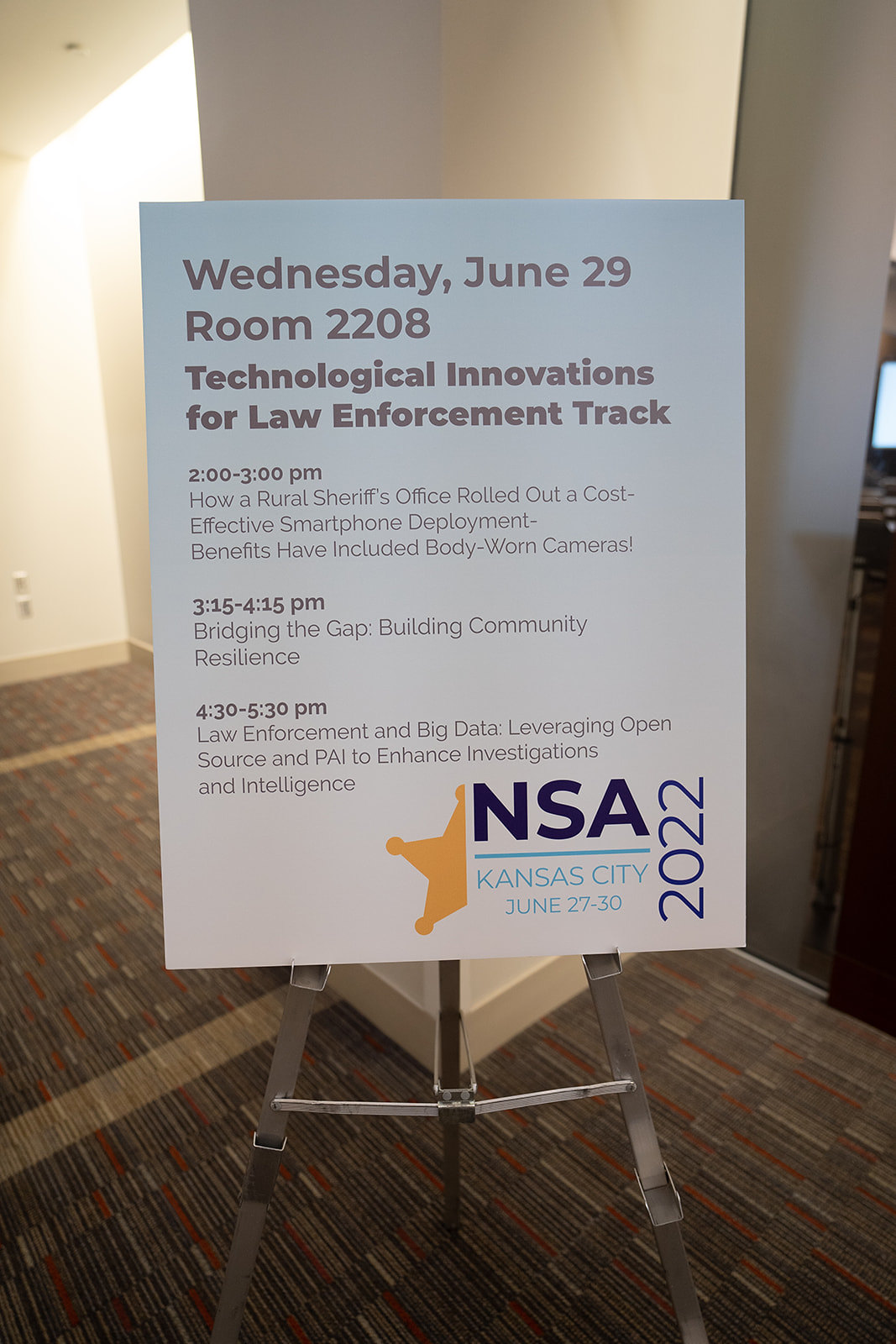This detailed photograph captures a large seminar poster stationed on a silver metal easel within a hallway, featuring a gray-striped carpet and gray walls. The prominently white poster is inscribed with gray text, detailing the schedule for the Technological Innovations for Law Enforcement Track seminar, set for Wednesday, June 29th, in room 2208. The schedule is as follows: from 2:00 to 3:00 p.m., a session on how a rural sheriff's office successfully rolled out a cost-effective smartphone deployment, enhancing its operations with body-worn cameras; from 3:15 to 4:15 p.m., a talk dedicated to bridging the gap and building community resilience; and from 4:30 to 5:30 p.m., a discussion on leveraging big data, open-source tools, and PAI to enhance law enforcement investigations and intelligence. At the bottom right of the poster, there's a gold logo of half a sheriff's star next to the text "NSA 2022, Kansas City, June 27-30." Near the poster, part of a seating area with a presentation screen is visible, suggesting the seminar’s intended setting.